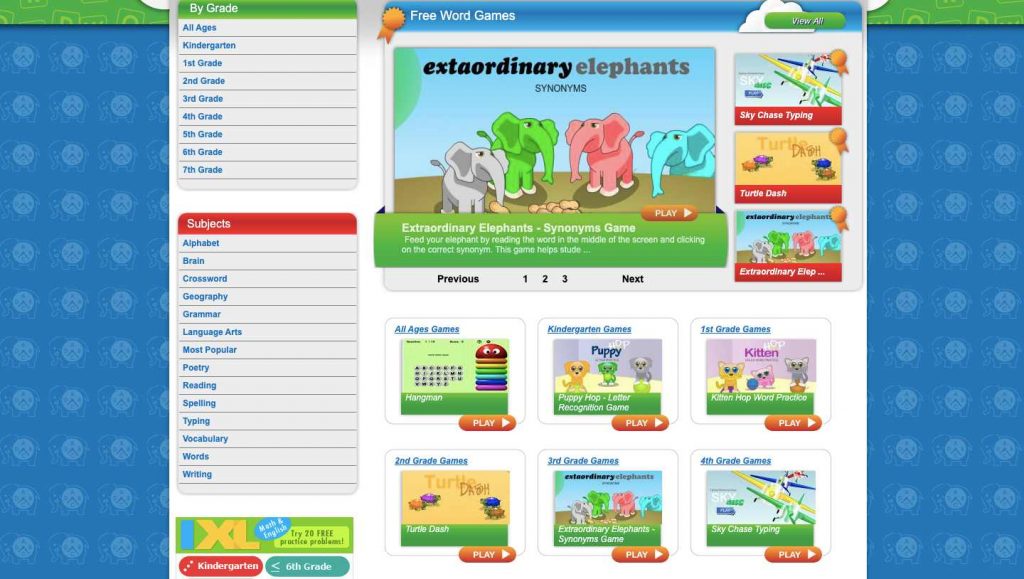This screenshot captures a vibrant, child-friendly website designed for gaming on a desktop or laptop PC, evident by its widescreen layout. The website's aesthetic is highly cartoonish, characterized by a blue background, rounded edges, and colorful illustrations, all of which contribute to its playful atmosphere. 

On the left side of the screenshot, a vertical column is divided into two sections: "By Grade" and "Subjects." The "By Grade" section features tabs for grades ranging from Kindergarten to 7th grade, allowing users to select their grade level easily. Below this, the "Subjects" section offers a variety of educational categories such as Alphabet, Brain Puzzles, Crosswords, Geography, Grammar, Language Arts, Poetry, and Spelling.

To the right of this column are images representing various games. The most prominent image features four elephants in different colors—gray, green, pink, and blue—standing together. This image is associated with a game titled "Extraordinary Elephants," though it's noteworthy that the word "Extraordinary" is misspelled as "Extraorinay" in the header above the elephants. However, a green banner below the elephants correctly spells "Extraordinary Elephants." This banner also labels the game as "Synonyms" and emphasizes it as a synonyms game.

Other visible game icons follow a similar colorful and cartoony design pattern, enhancing the overall engaging and educational experience for children.